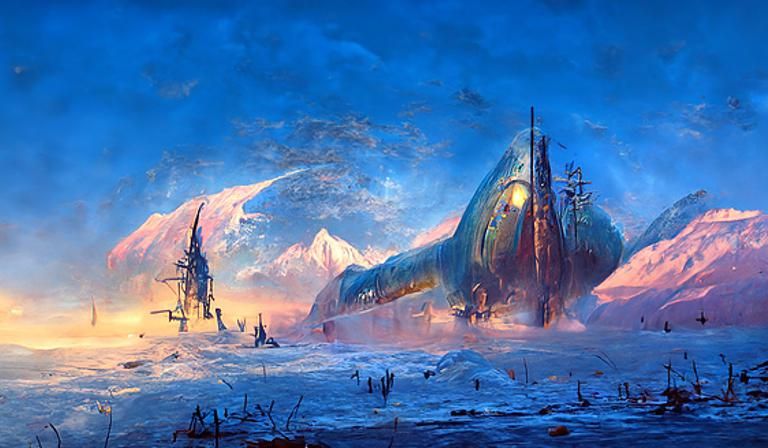The artwork is an ethereal, pastel-themed painting that blends elements of fantasy and sci-fi. It depicts a brilliant blue sky with faint white and gray clouds, beneath which lie majestic, snow-capped mountains in the backdrop. The mountains have a pinkish hue, suggesting the soft glow of a setting sun. Below the mountains, a large blue ocean with white cresting waves stretches across the scene, dotted with debris and parts of sunken ships.

In the center of the ocean rises a massive, enigmatic metal object, reflecting light and evoking the appearance of a futuristic submarine or battleship. Flanking this imposing structure are smaller objects, including a tall tower with numerous appendages and a ship that resembles a destroyer. The overall atmosphere of the painting is dark and dreamy, heightened by the contrasting shades of blues, blacks, and the pinkish highlights of the setting sun.

Adding to the fantastical quality are the tall trees emerging from the water, their forms obscured by a pink haze that complements the sunset. The image conveys a surreal, almost otherworldly landscape where nature, destruction, and technology interplay in a hauntingly beautiful setting.